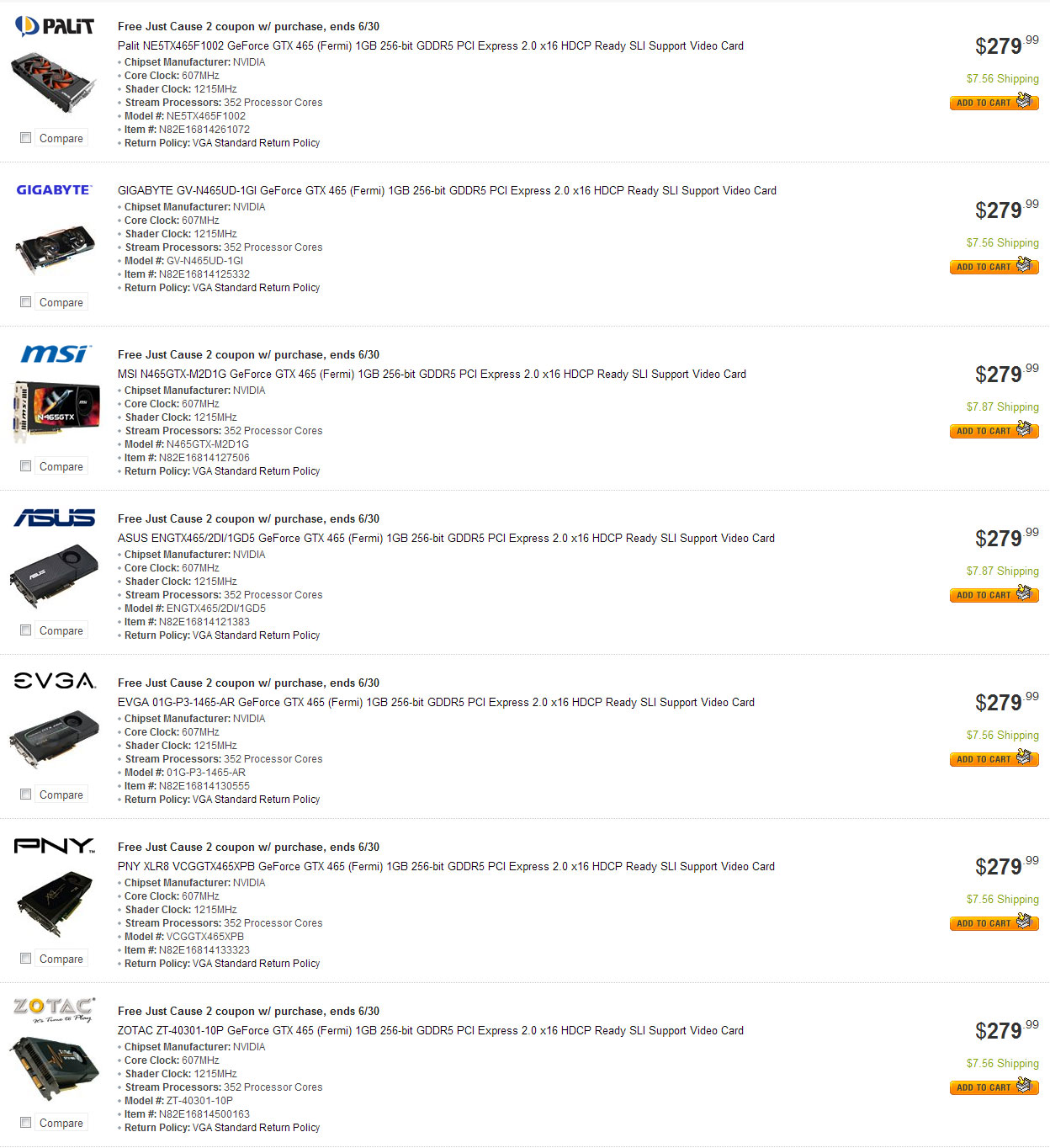The image displays a pricing comparison table against a white background, with thin blue lines separating each item for clarity. At the top left, there is a palette icon accompanied by a blue and yellow insignia. Beside it is an image of a product priced at $279.92, along with an orange "Add to Cart" button. The subsequent entries are as follows:

1. Gigabyte: Priced at $279.99 with an orange "Add to Cart" button.
2. MSI: Priced at $279.99 with an orange "Add to Cart" button.
3. Asus: Priced at $279.99 with an orange "Add to Cart" button.
4. EVGA: Priced at $279.99 with an orange "Add to Cart" button.
5. PNY: Priced at $279.99 with an orange "Add to Cart" button.
6. ZOTAC: Priced at $279.99 with an orange "Add to Cart" button.

Each item is clearly marked with its brand and price, and all except the first are aligned in a similar format for easy comparison.